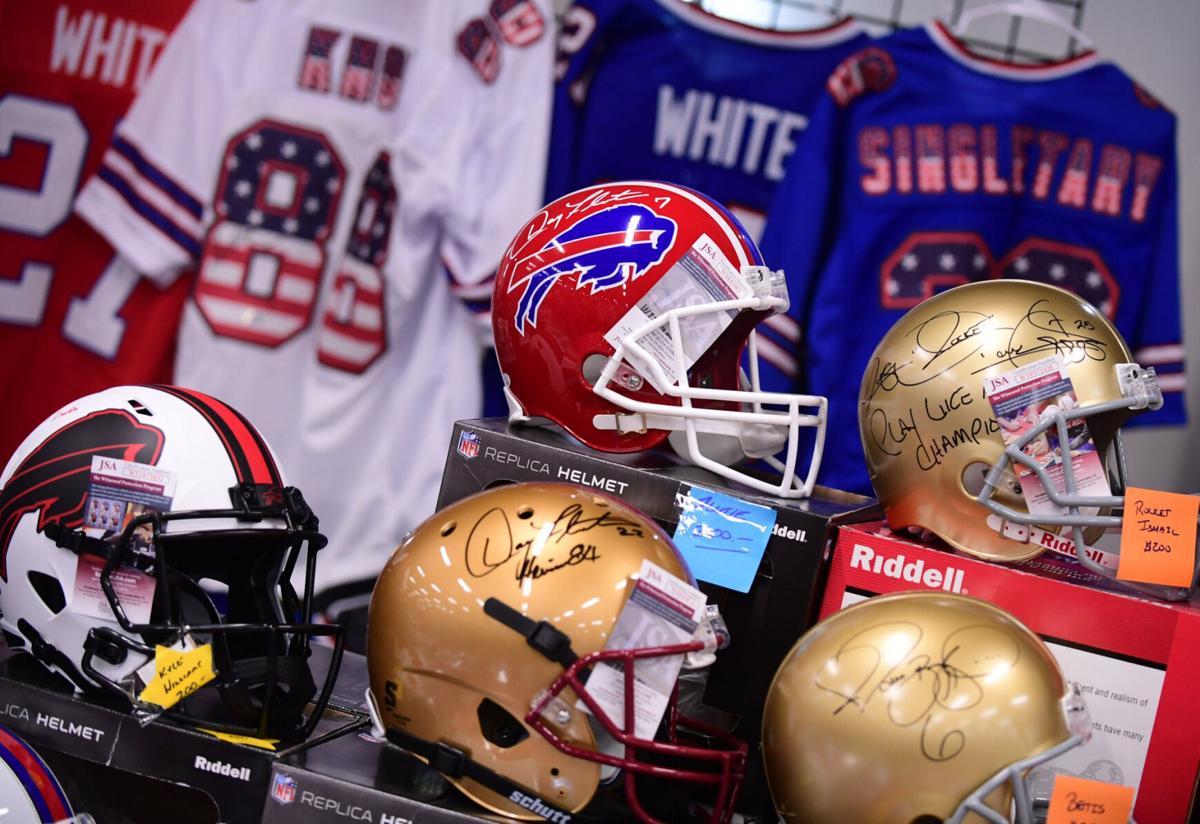The image depicts a collection of American football memorabilia, prominently featuring five miniature football helmets and four jerseys displayed in the background. Among the helmets, three are gold-colored without logos but bearing signatures from players, signifying their autographed nature. The remaining two helmets represent the Buffalo Bills: one is predominantly red with a blue buffalo design and a red stripe, while the other is white with a red stripe across the top and a black-outlined buffalo symbol with red accents. The jerseys, hung on hangers, span a color scheme of blue, white, and red. Notably, one jersey is red with white writing and numbering, another is white with a distinct American flag theme integrated into the number "88," and two others are blue, trimmed with red and white. These blue jerseys also feature an American flag theme in the numbers and names, with one likely bearing the name "Singletary." Each jersey is adorned with a player's number and name, enhancing their collectible appeal. The setup and accompanying pamphlets suggest a setting possibly tied to a charity auction or a memorabilia display.